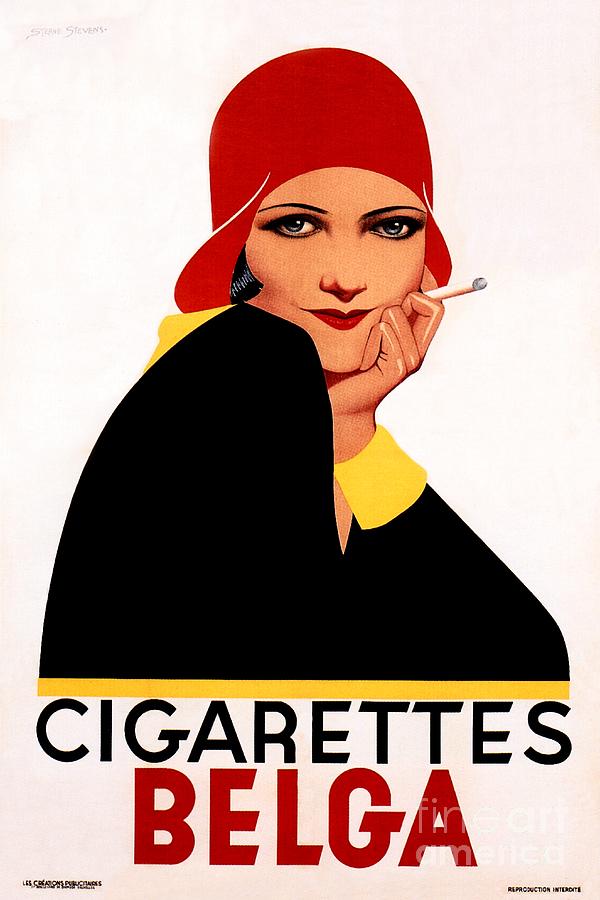This is a color image of an old advertisement poster, likely from the 1920s, depicting a stylish woman smoking Belga cigarettes. The poster features a light pinkish background reminiscent of aged paper. The woman, drawn in a vintage style, is facing slightly to the right, with her right shoulder visible and her left hand resting under her cheek while holding a cigarette. She has short, black hair combed towards her cheekbones, partially hidden by a large red hat with flaps on either side, characteristic of 1920s fashion. 

She is adorned in a black dress with distinct yellow cuffs. Her striking appearance is highlighted with red lipstick, dark eyebrows, and grayish-blue eyes. Beneath her image, a bold yellow line runs horizontally, above the large black lettering that reads "CIGARETTES," with "BELGA" in even larger red letters beneath it. Some blurred French text appears at the top left and additional small black writing is located at the bottom corners of the poster, though it is too small to discern. The word "REPRODUCTION INTERDITE" suggests that the poster reproduction is prohibited.